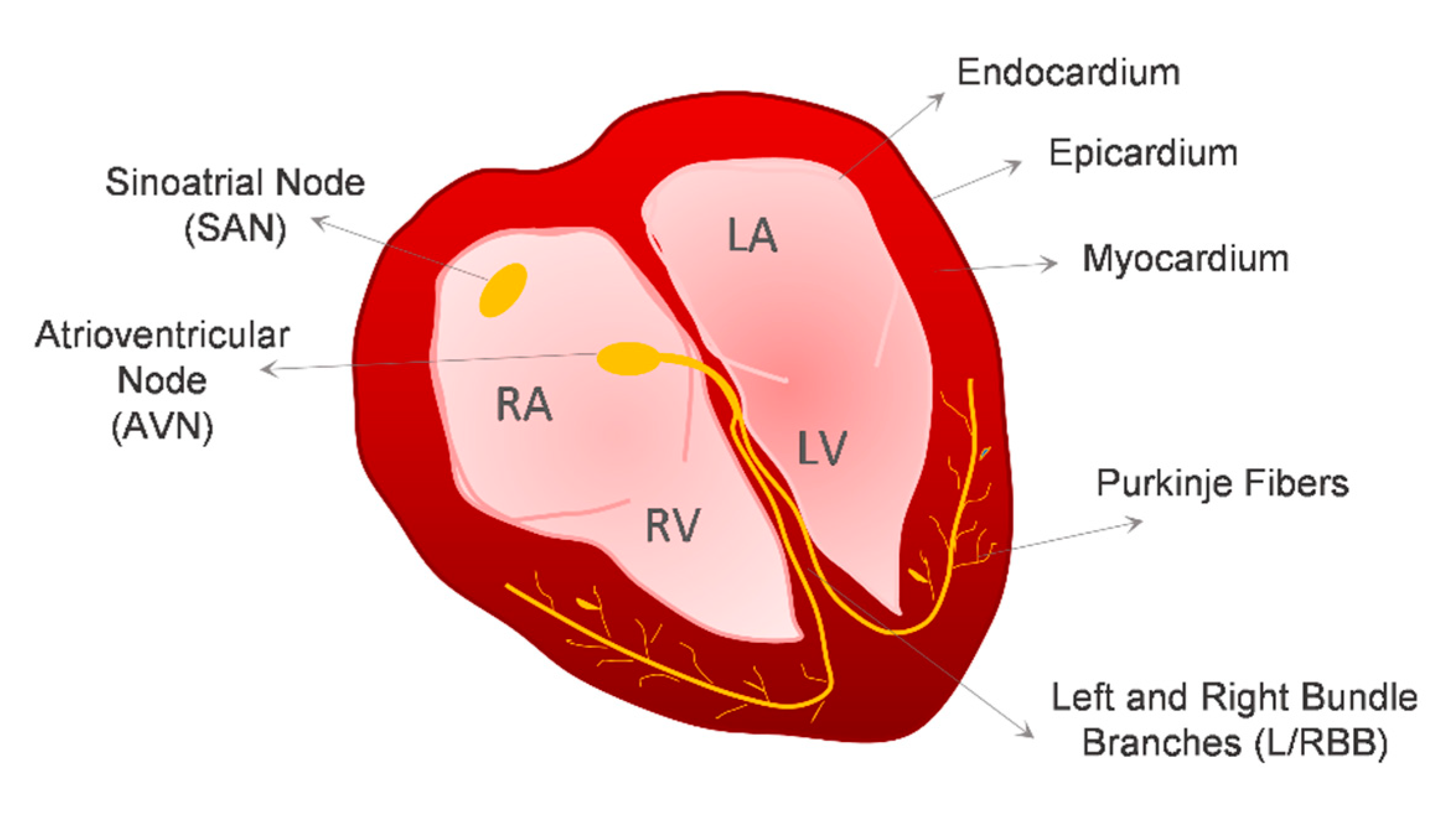This anatomical drawing is a simple, yet detailed illustration of the human heart, colored in red. Key structural elements and layers are labeled with annotations and arrows pointing to specific parts. The heart features a branching yellow vein-like structure through the center. It is divided into four chambers, labeled with small gray text: RA (right atrium) at the top left, RV (right ventricle) below that, LA (left atrium) on the top right, and LV (left ventricle) below it. Around the heart, starting from the top right and moving clockwise, labels include: endocardium, epicardium, myocardium, Purkinje fibers, left and right bundle branches, atrioventricular node, and sinoatrial node. This detailed labeling provides clear insight into the heart's anatomical and functional aspects.